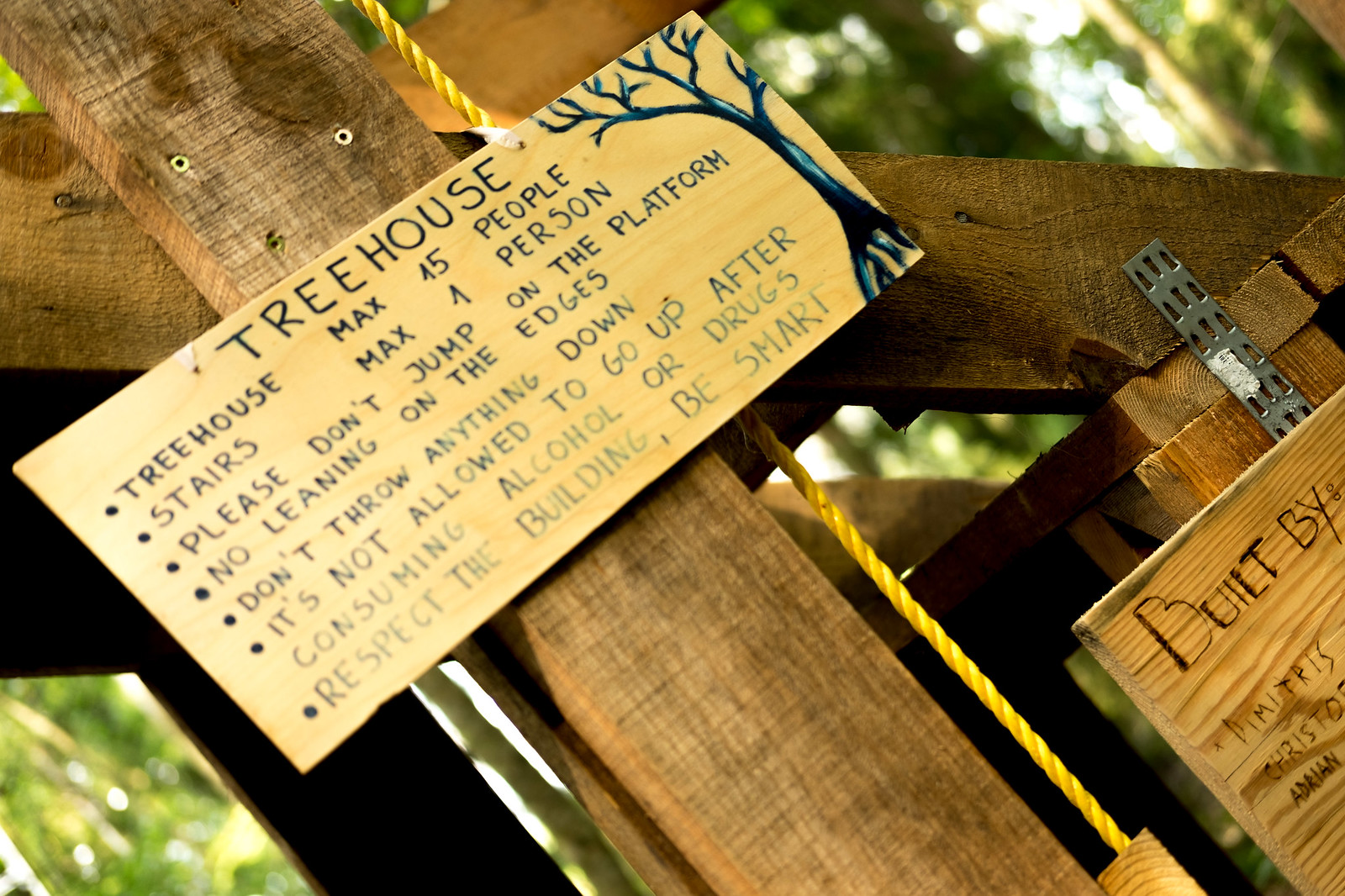In the image, we see a close-up perspective of a rustic, wooden treehouse, adorned with a prominently displayed sign bolted to several wood beams, with one beam extending vertically and another horizontally across. The sign, written in black text, lays out various rules and guidelines for visitors. 

It reads: "Treehouse, max 45 people. Stairs, max one person. Please don't jump on the platform. No leaning on the edges. Don't throw anything down. It's not allowed to go up after consuming alcohol or drugs. Respect the building, be smart." This detailed information is organized into bullet points and accompanied by an illustration of a tree, etched in black with a touch of blue. 

Additionally, there is another wooden plank, slightly cut off in the image, which states "built by," but the name is not legible. The background reveals blurred green foliage, indicating that the treehouse is situated outdoors amidst lush greenery, integrating seamlessly with its natural surroundings. Visible screws and a steel connector hold the wooden boards together, highlighting the treehouse's handcrafted construction.